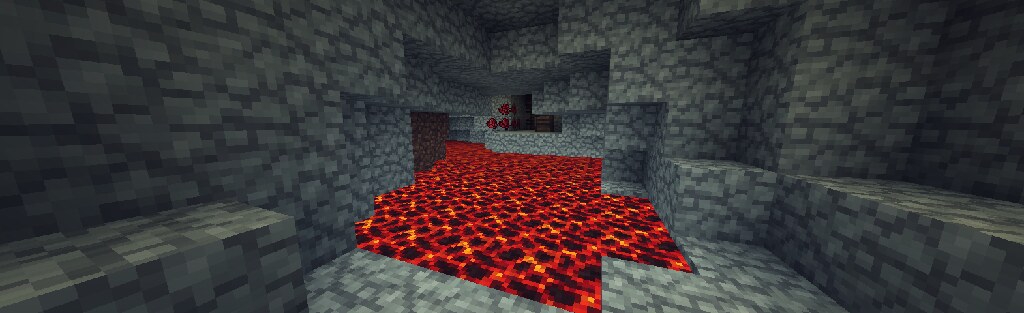This super widescreen screenshot from the game Minecraft captures an intricately detailed interior layout of a dimly lit cave. The scene is constructed entirely from the game's signature stylistic blocks, prominently featuring rugged cobblestone blocks that define the cave's structure. The cave floor is interspersed with glowing red and black blocks, simulating the presence of lava and adding an ominous illumination to the scene. In the background, several blocks appear to contain various minerals, hinting at the potential rewards for players who choose to mine in this subterranean environment. The image is heavily vignetted on the left and right edges, deepening the sense of enclosure and darkness appropriate for a cave setting.